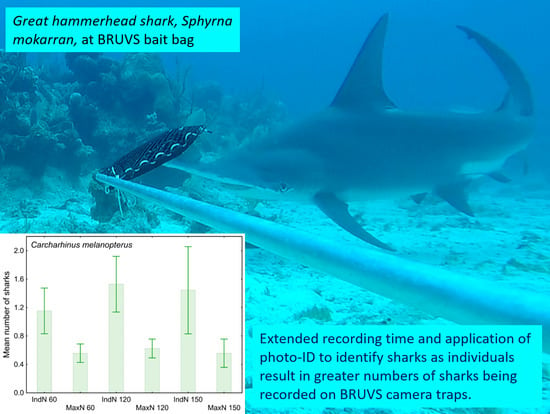The underwater photograph showcases a majestic Great Hammerhead Shark (Sphyrna mokarran), gracefully gliding above a seabed of light-colored sand and coral-like plant life. The scene is set in clear, blue water with ample lighting that highlights the shark's distinctive T-shaped head, large fins, and gray body with a white underside. At the bottom of the image, a lengthy metallic rod extends into the frame, ending in a black netted object identified as a "Bait Bag" used for scientific studies to attract sharks.

In the upper left corner, a light blue text box with black font reads "Great Hammerhead Shark (Sphyrna mokarran) at B-R-U-V-S Bait Bag." In the lower right corner, another light blue text box provides information about the scientific study, stating, "Extended recording time and application of photo ID to identify sharks as individuals result in greater numbers of sharks being recorded on B-R-U-V-S camera traps."

Additionally, the lower left corner of the image features a vertical bar chart in a sea green color against a white background, bordered by a black box. The y-axis, labeled "mean number of sharks," ranges from 0.0 to 2.0 in increments of 0.4, while the x-axis lacks a descriptive key but alternates between "INDN" and "MAXN" with numerical values of 60, 120, and 150. The chart aims to visualize the shark population data collected during this research study.